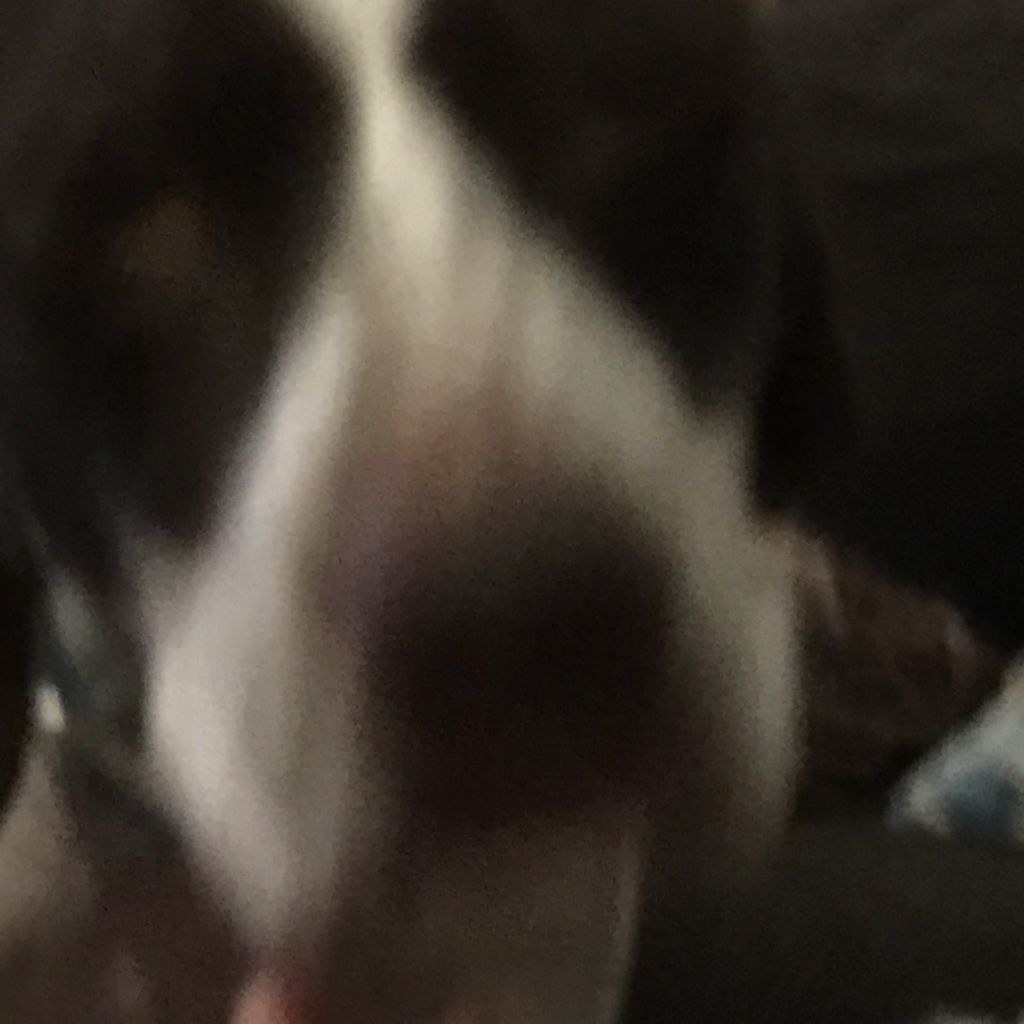This photograph, while blurry, captures the face of a dog. The image reveals the dog's black nose prominently, alongside a white portion on its face. The dog's tongue seems to be sticking out, and the reflective, glowing effect in its eyes, similar to how pets' eyes look in low light, is visible. The dog has black markings around its eyes and a distinctive white streak running from its nose up between its eyes. In the grainy background, some discernable features include what appears to be a tan piece of furniture. Atop this furniture, there are two objects: one white and one tan. The overall image, despite its blurriness, provides a glimpse of the dog's unique facial features and the surrounding environment.